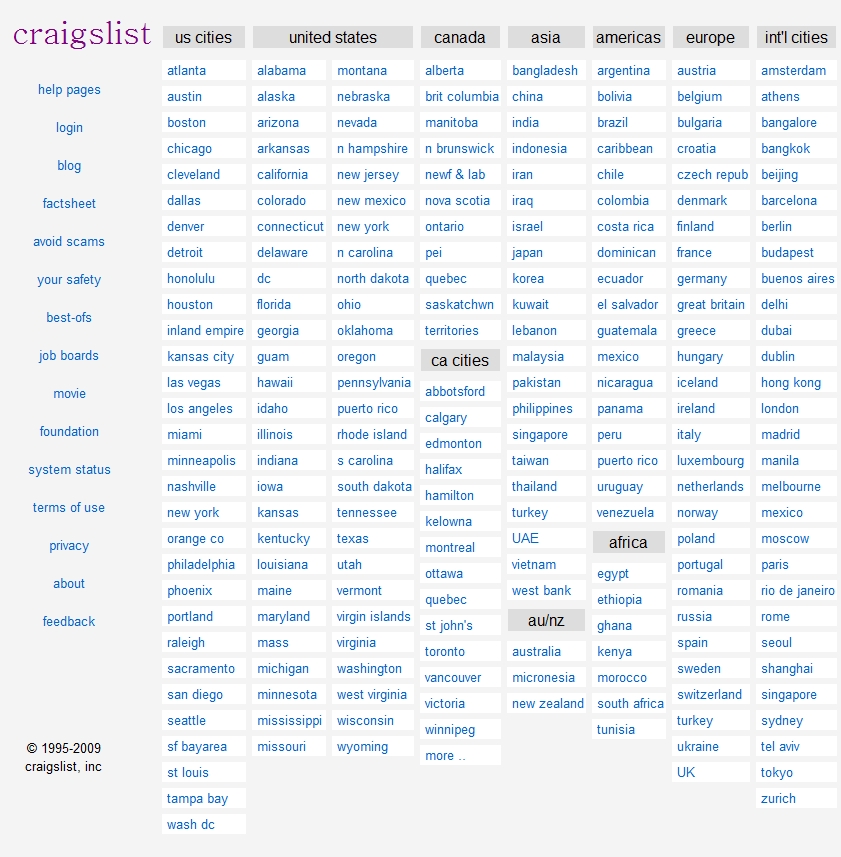The image features a minimalist grey background. In the top left corner, displayed in lowercase purple letters, is the word "craigslist." Along the entire left side of the image runs a vertical column listing various sections from top to bottom, including: "help pages," "login," "log," "fact sheet," "avoid scams," "your safety," "best ofs," "job boards," "foundation," "system status," "terms of use," "privacy," "about," and "feedback." At the bottom of this column, it notes "copyright 1995-2009 craigslist incorporated."

At the very top of the image, from left to right, there's a horizontal menu with categories: "U.S. cities," "United States," "Canada," "Asia," "America," "Europe," and "international cities." Below this, a secondary column on the left lists U.S. cities, starting with "Atlanta," followed by "Austin," "Boston," "Chicago," "Cleveland," "Dallas," "Denver," "Detroit," "Honolulu," "Houston," "Inland Empire," "Kansas City," "Las Vegas," "Los Angeles," "Miami," "Minneapolis," and concluding with "Nashville."